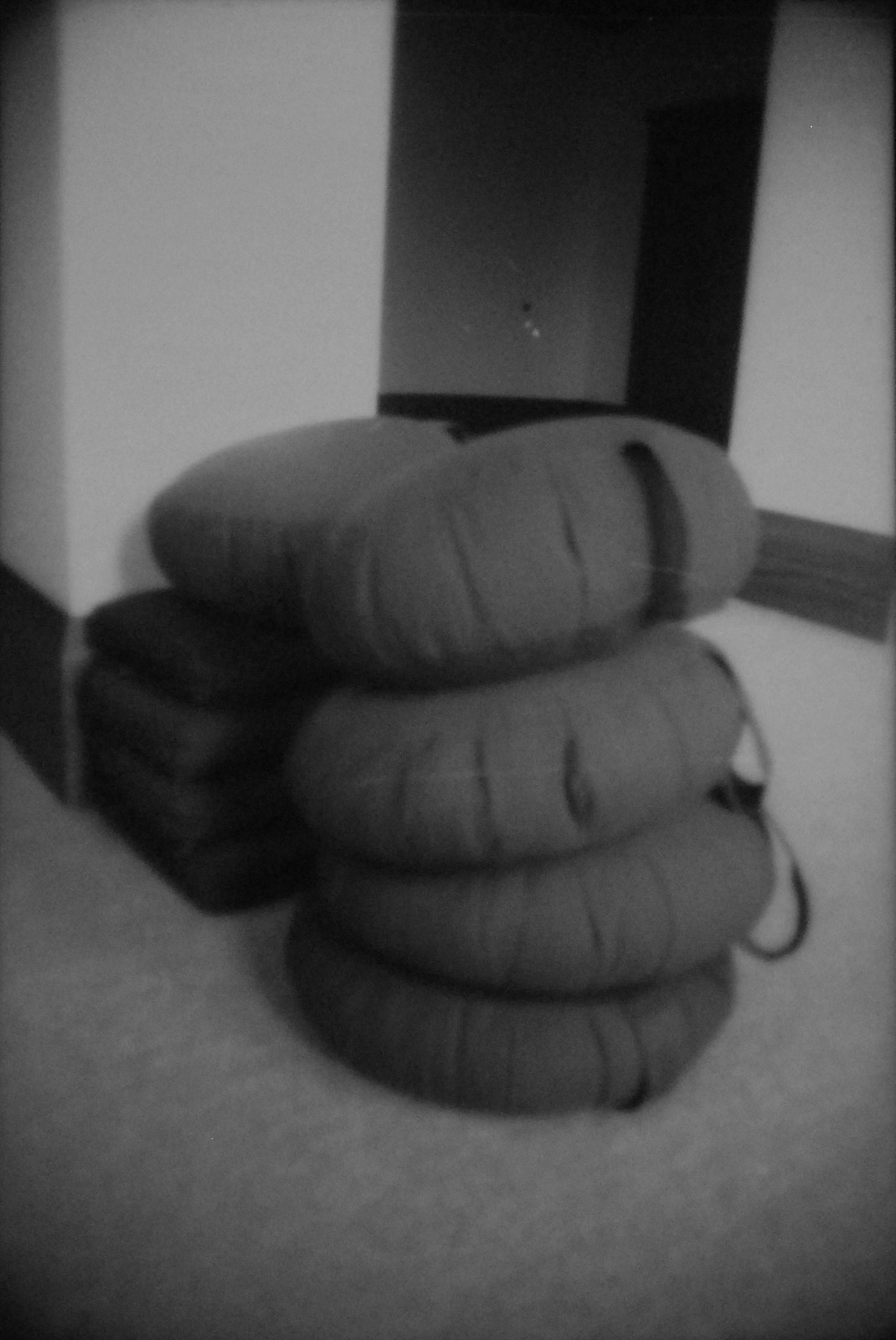This is a black-and-white digital photograph depicting a somewhat blurry stack of rounded, gray cushions with handles or black straps, arranged in an indoor setting. In the center of the image, four of these rounded cushions are neatly piled atop each other on a tan-colored carpet. To the left, another round cushion rests on top of a few dark gray, rectangular cushions. The background features white walls, a tall running board with a grayish wood color at the base, and a darker doorway that recedes into the shadows, suggesting low lighting conditions behind it. The floor appears to be carpeted, with edges that show a darker tinge. The edges of the cushions have gathered lines, adding texture to their appearance. The overall scene is devoid of any other objects, creating a focused composition on the stacked cushions.